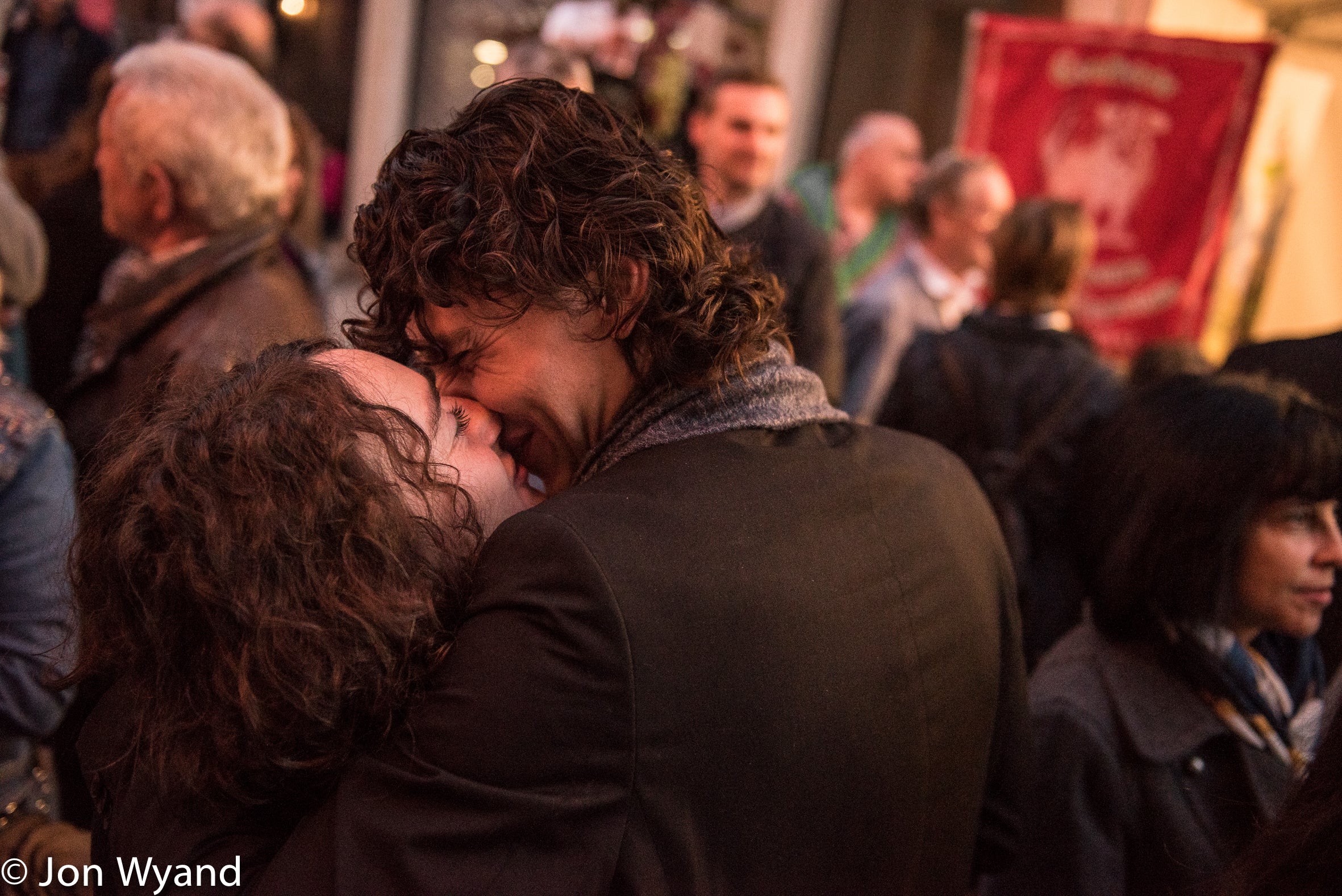In the center of the photo, a man and a woman are tenderly kissing and holding each other amidst a crowd. The man, appearing to be in his 30s, stands taller than the woman and has long, wavy brown hair that falls past his ears and over his shoulders. He is dressed in a dark brown sport coat and a light brown scarf. The woman has medium-length, dark brown curly hair and is similarly smiling and kissing the man. While their embrace takes up most of the focus, you can see other people blurred in the background, including a guy wearing a green shirt or jacket and an older man with gray hair and a brown jacket in the upper left. In the lower right, a moderately dark-skinned woman with medium black hair is looking off to the right. Part of another head and arm, possibly of the woman's parent, is visible to the left. A red silk or satin banner with a white dog shape hangs from the upper right corner. At the bottom of the image, the copyright symbol followed by "GON WYAND" is visible in white letters, possibly indicating the photographer.